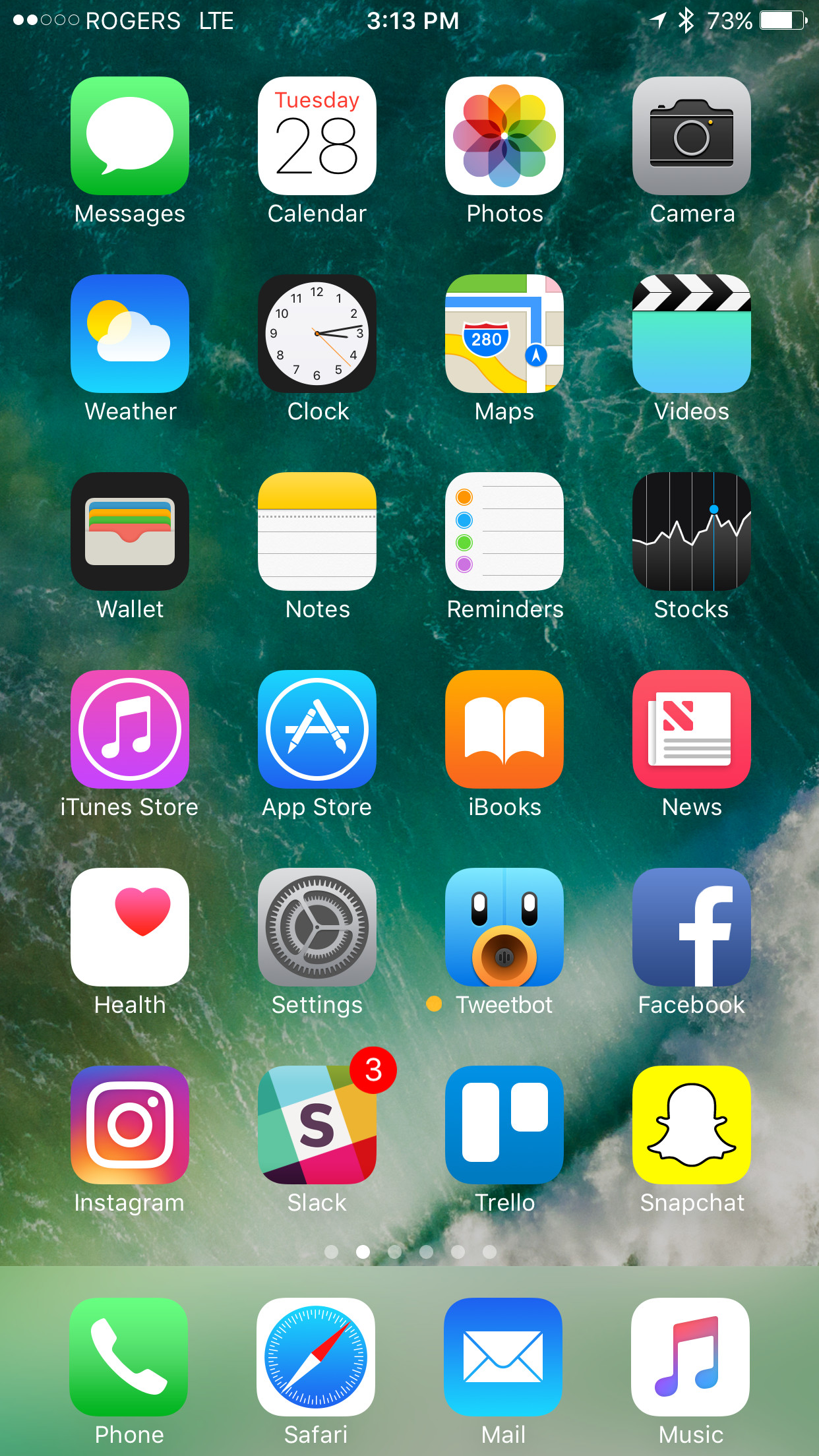The image showcases the screen of a mobile device, likely a phone or a tablet, identifiable by the status bar at the top displaying "Rogers LTE," the current time, and battery life. The background is a serene, greenish-blue depiction of ocean water, adding a tranquil aesthetic to the interface. Below the status bar, a series of diverse widgets are neatly arranged. These include a clock widget, and icons for various apps like Photos, Snapchat, and Instagram. At the very bottom, the main dock is subtly grayed out, featuring icons for key applications: Phone, Safari, Mail, and Music. Each icon includes a representative image, ensuring easy identification of each function. The overall layout is clean and visually appealing, blending functional app shortcuts with an inviting oceanic backdrop.